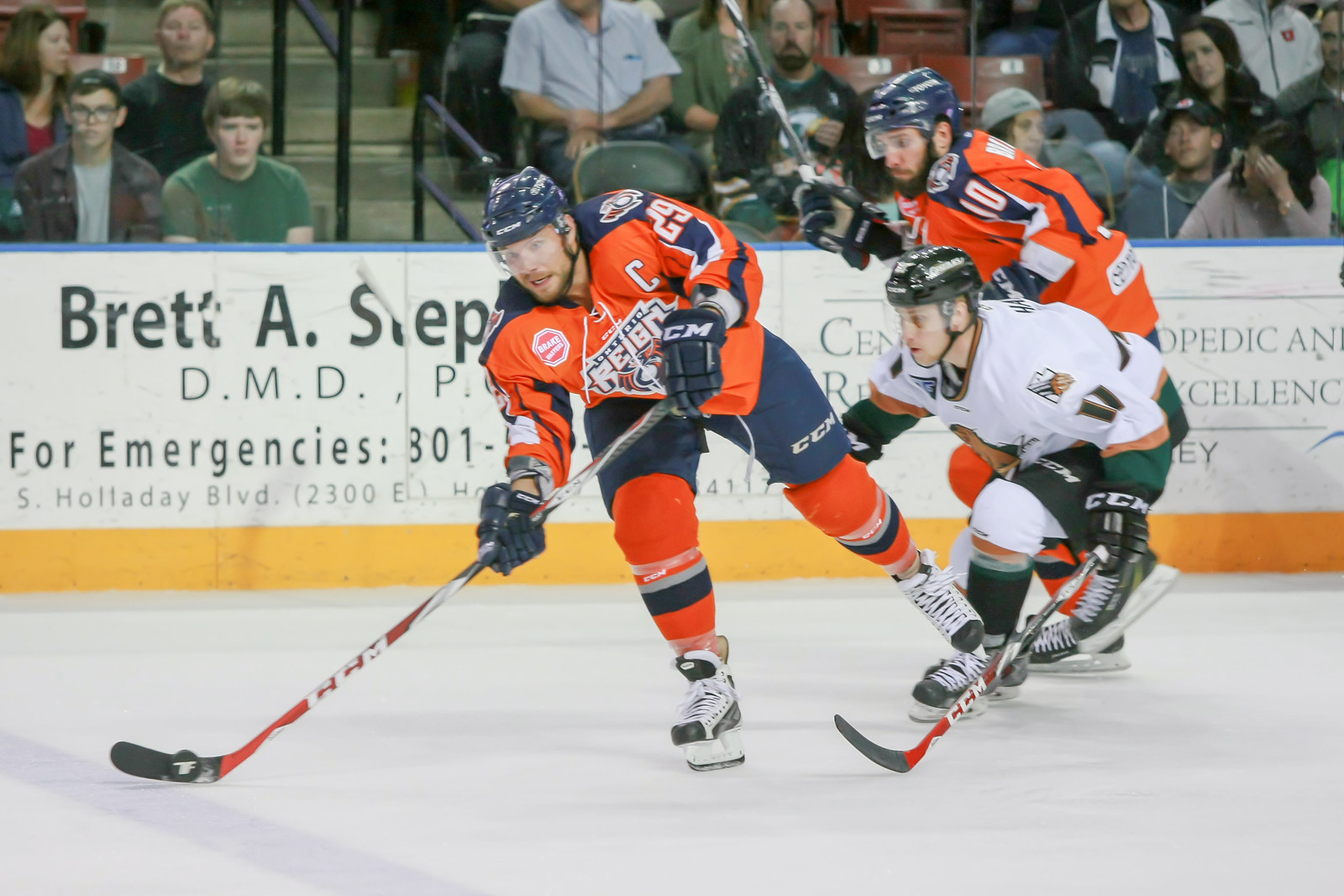The image captures an intense moment from a live hockey game, with three players in focus on the ice. Two of the players are dressed in orange and blue uniforms, representing what seems to be the Ontario Rain team, complete with blue helmets, white and black ice skates, and hockey sticks colored orange and black. The player on the far left has the puck on their stick, appearing ready to either guide or shoot it. Close to them, to the right, is an opponent in a white jersey with green and gold trim and a dark green helmet. The opponent's skates are also dark green with white blades. Another player from the Ontario Rain team stands behind the opponent, raising their hockey stick in the air with their right hand, as if preparing to intercept or assist. Behind the players, a crowd of spectators watches intently through the protective glass. Above the crowd, a white banner with bold black and grayish text advertises a business, with partially visible details including "Brett A. S., DMD" and "For Emergencies 301 S. Holiday Blvd 2300." The scene is a snapshot of the dynamic and competitive energy typical of a live hockey game.